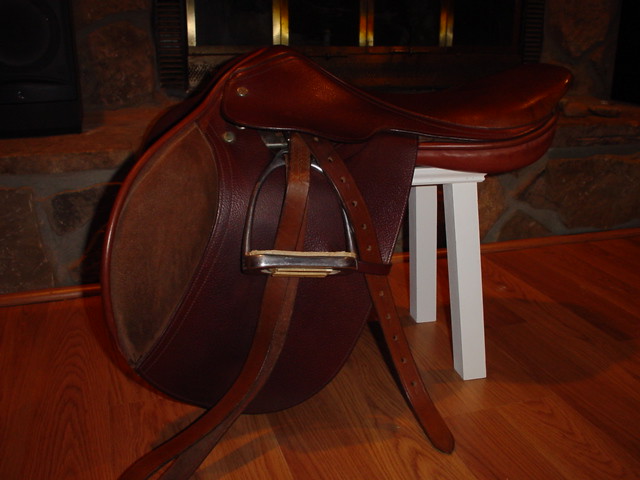This detailed image depicts a deep reddish-brown leather saddle, intricately crafted and well-maintained, resting prominently on a small white stool. The setting appears to be indoors on a wooden surface, possibly a table or stage, which matches the saddle's rich hue but is slightly lighter in tone. The saddle features numerous leather straps, some resembling belts with adjustable holes, and has metal attachments, likely stirrups, on either side. A large opening at the front suggests it fits around a horse's neck. The background includes a brick wall with windows, adding to the neutral lighting of the scene, hinting at a possible showcase or display within a building. This meticulously designed saddle, with its prominent large buttons, showcases both its aesthetic craftsmanship and functional purpose.